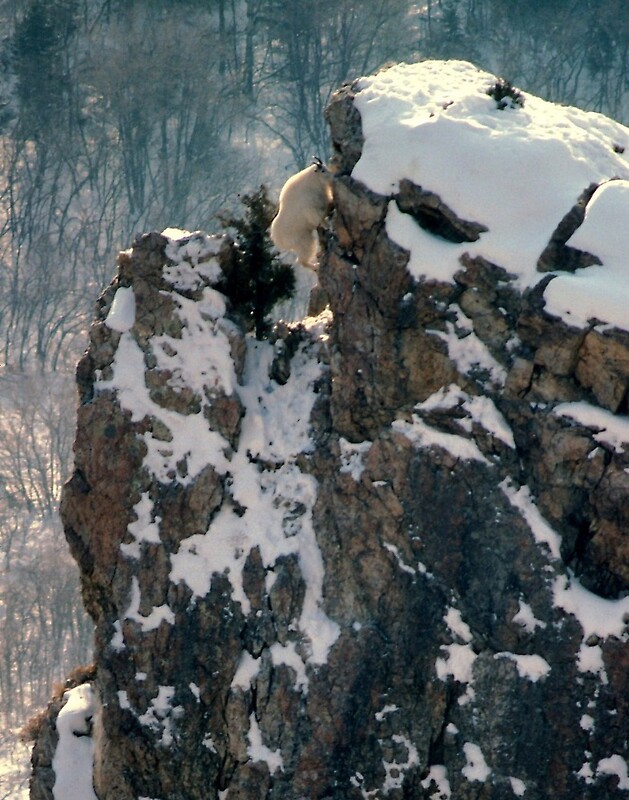In this breathtaking image, a majestic mountain peak stands proudly covered in pristine snow. The snow-capped summit glistens under the sunlight, contrasting beautifully with the dark, rugged terrain of the mountain. Surrounding the base of the mountain, a lush valley can be seen, adorned with verdant green trees that add a touch of life to the serene landscape. Scattered across the lower slopes of the mountain are additional patches of dense trees, creating a picturesque mosaic of white, green, brown, and black hues. Remarkably, a lone tree and a determined shrub have managed to take root even near the summit, showcasing nature's tenacity. The image, free of any text, captures the raw beauty and tranquility of this mountainous region.